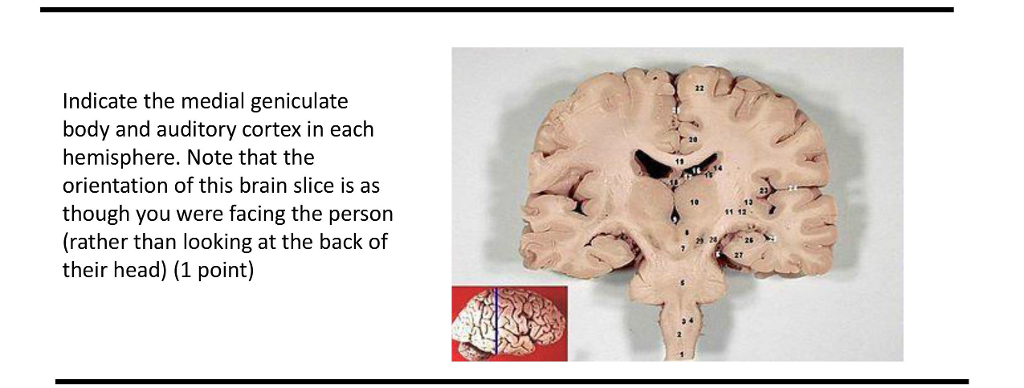This image appears to be a detailed, textbook-style illustration from a medical or educational source, featuring both text and photographs. On the left-hand side, the text reads: "Indicate the medial geniculate body and auditory cortex in each hemisphere. Note that the orientation of this brain slice is as though you are facing the person rather than looking at the back of their head." This explanatory note is crucial for properly understanding the orientation of the brain slice. To the right, there is a labeled display of a brain slice that resembles a vertically cut piece of cauliflower, with distinct numbered points indicating various brain regions. Below this main image is an inset showing a complete brain, marked with a line, possibly purple, that indicates the location of the brain slice shown in the main image. This line serves as a guide to understand where the section was taken from in the context of the whole brain. The combination of these elements provides a comprehensive view designed to aid in identifying specific parts of the brain, likely for educational or preparatory purposes.